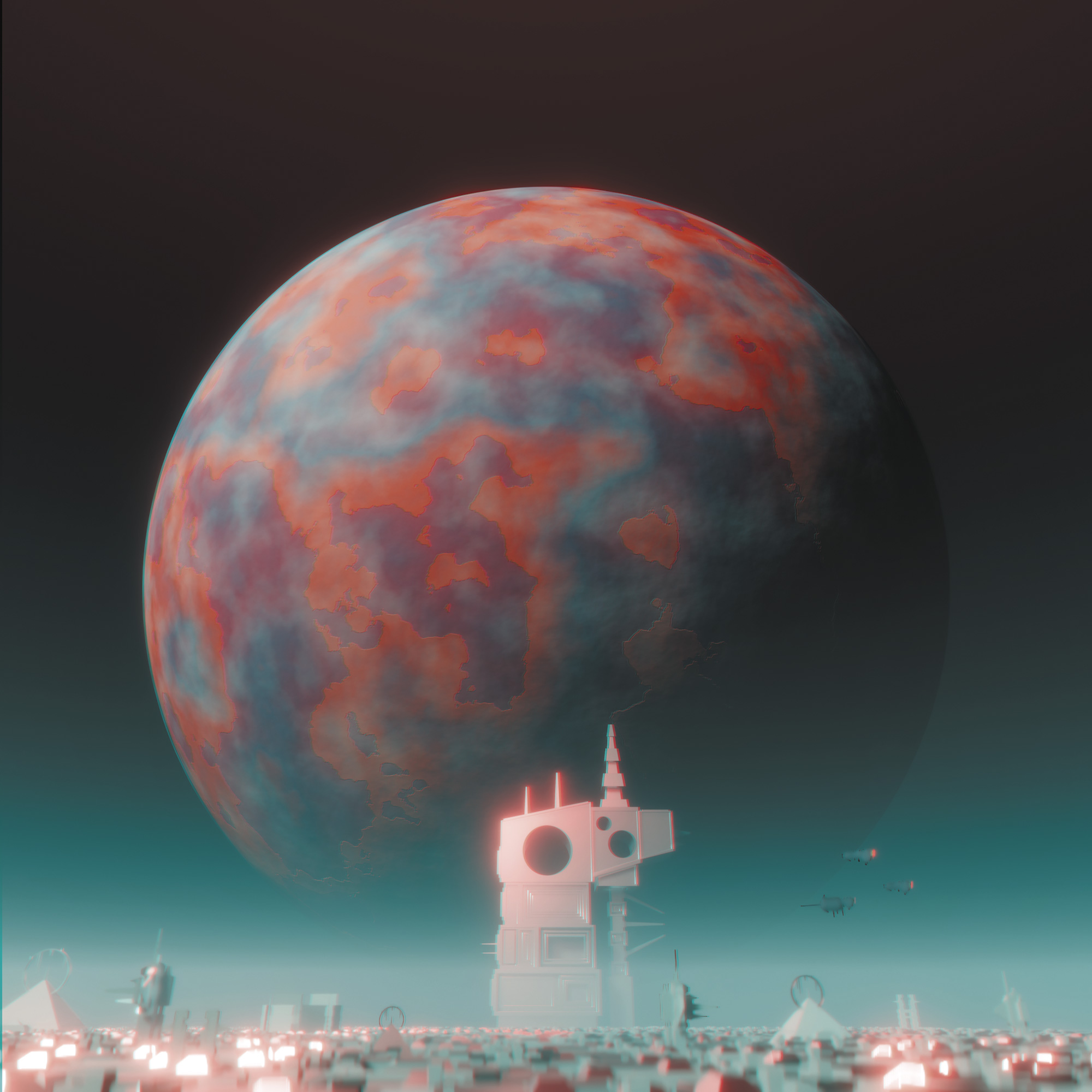The image depicts a futuristic or alien cityscape set against a majestic space backdrop. Dominating the scene is a large, round planet, primarily blue and purple with patches of red and gray, suggesting varied landmasses or gaseous formations. The planet occupies the center of the image, hovering against a dark sky that fades into a misty teal gradient towards the surface. In the foreground, there's an illuminated white structure, possibly a space station or towering building with circular openings and intricate designs. Surrounding this main structure is a sprawling city of smaller buildings, some with antennas, others resembling tents or small homes, all interspersed with bright lights. Three small flying vehicles are visible near the right side of the towering structure, while a robot and a couple of pyramids can be seen on the ground to the left. This detailed digital artwork captures a vivid and otherworldly atmosphere.